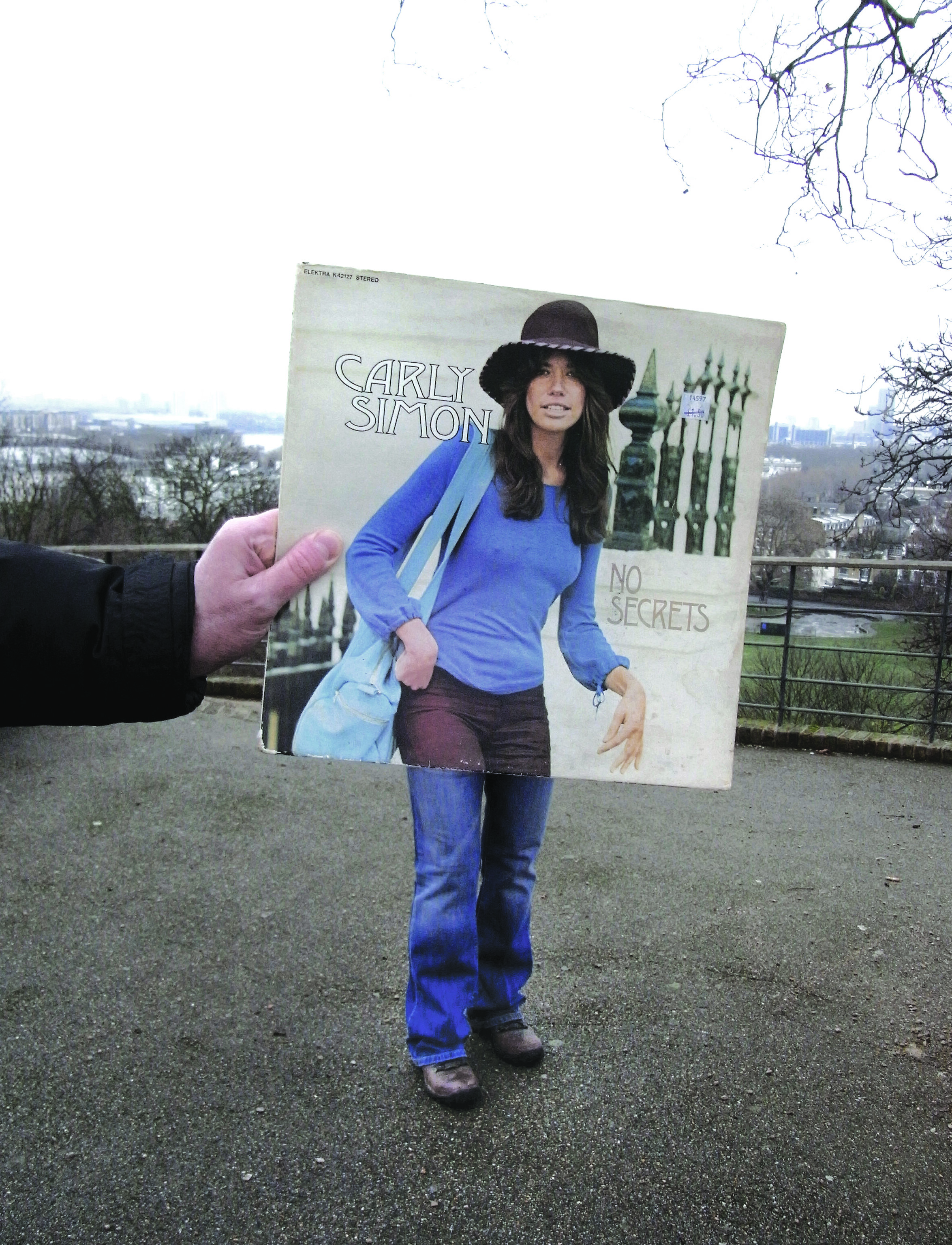In this clever and detailed photograph, a woman is positioned centrally, standing on an asphalt surface with a cityscape visible in the background. She is wearing blue jeans and brown shoes. In front of her, a man's hand, clad in a black jacket, holds up a Carly Simon album cover titled "No Secrets." The album cover is aligned precisely with the woman's lower body, giving the illusion that Carly Simon's image continues seamlessly from her waist down. Carly Simon, depicted on the album cover, is wearing a blue shirt, brown or purple pants, a brown hat, and carrying a blue bag. The fusion of the album cover with the woman's real-life jeans creates a playful mimicry of Carly Simon's iconic look, making it appear as if Simon herself is part of the scene.